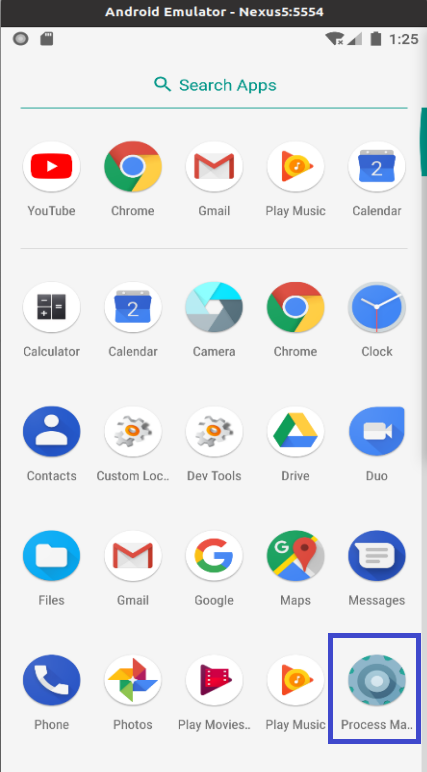This image showcases a screenshot of an Android Nexus 5 emulator with the model number 5554. At the very top of the screen, various status icons are displayed, including indicators for Wi-Fi signal strength, network signal strength, battery level, and the device's time, which shows as 1:25. Below these icons is a search bar labeled "Search apps."

The main area of the screen is populated with various app icons arranged in a grid layout. The apps visible include YouTube, Chrome, Gmail, Play Music, Calendar, Calculator, Camera, Clock, Contacts, Custom Lock, DevTools, Drive, Dual, Files, Gmail (again), Google, Maps, Messages, Phone, Photos, Play Movies, Play Music, and Process Manager. Notably, the Process Manager app, located in the bottom right corner, is highlighted in blue, indicating it has been selected or is currently active. The clean, organized interface represents a typical app screen of an Android device emulator.